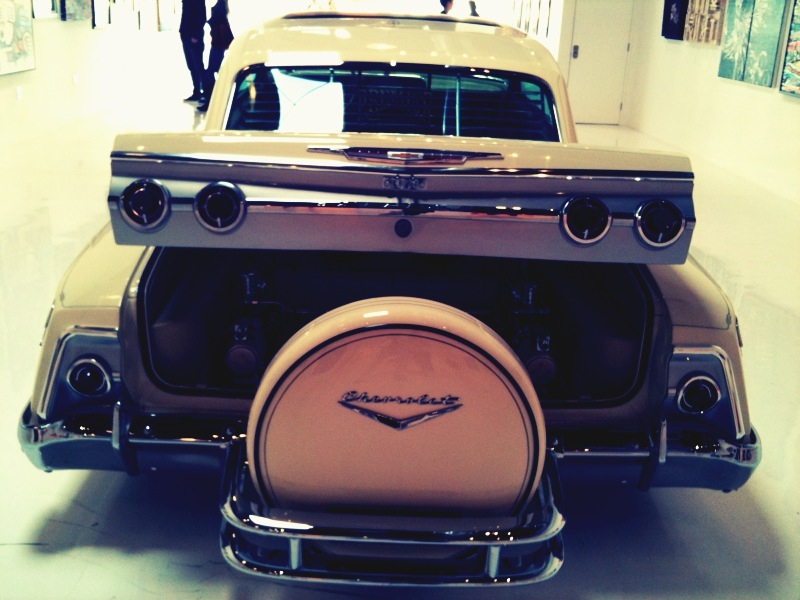The image showcases a striking classic Chevy Chevelle, resplendent in a unique combination of white, cream, and pink hues, with its trunk popped open. The scene is set inside what appears to be a showroom or an art gallery, further accentuating the car's vintage charm amidst an artistic backdrop. A chrome rear bumper adorned with four circular taillights and an extra wheel case attached to the trunk underscores the vehicle's classic aesthetic. The trunk proudly displays the Chevrolet emblem. In the background, four people can be seen, albeit partially obstructed, observing the Chevelle and the surrounding art pieces, adding to the dynamic atmosphere of the setting. The overall ambiance of the image conveys a blend of automotive nostalgia and artistic appreciation, capturing the attention of onlookers at this auto show/gallery.